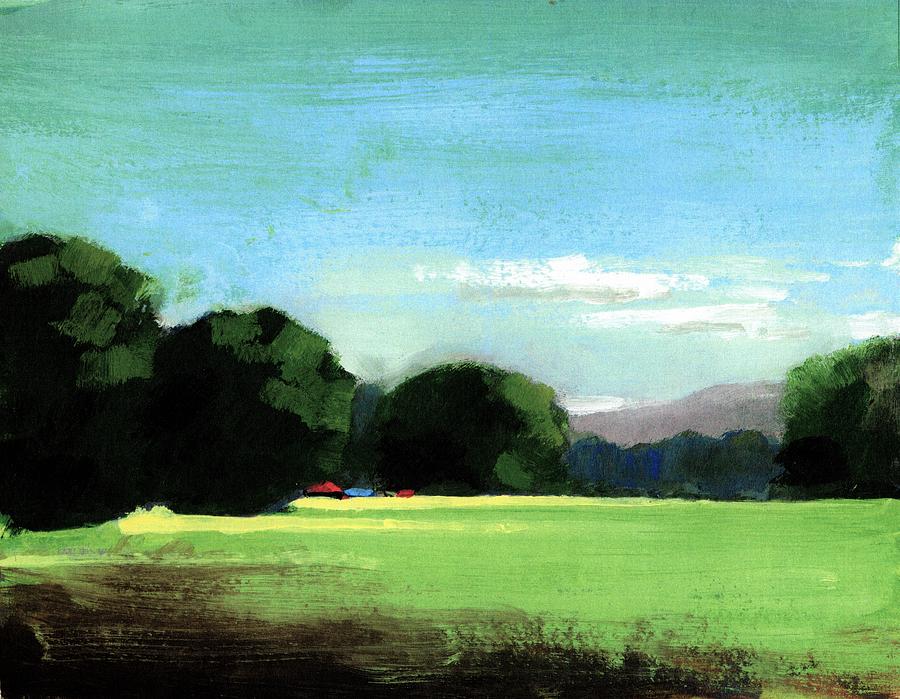This painting presents an abstract and simplistic outdoor scene, with a rustic charm. The sky occupies the top third of the canvas, painted in a blend of blue with brush strokes of white clouds, interspersed with streaks of green at the very top. The middle section features large, round clumps of trees or bushes, primarily positioned towards the left but with one to the right. Behind these trees, there is a subtle depiction of a gray mountain ridge. The foreground is a green field, accented with quick, horizontal streaks of yellow, suggesting grass. The very bottom of the painting contains rough, dark brown swaths of paint, providing a strong base to the composition. Adding a touch of mystery, red and blue objects appear near the trees, their identities unclear. The painting's overall abstract nature and minimalistic color palette give it a serene, yet intriguing feel.